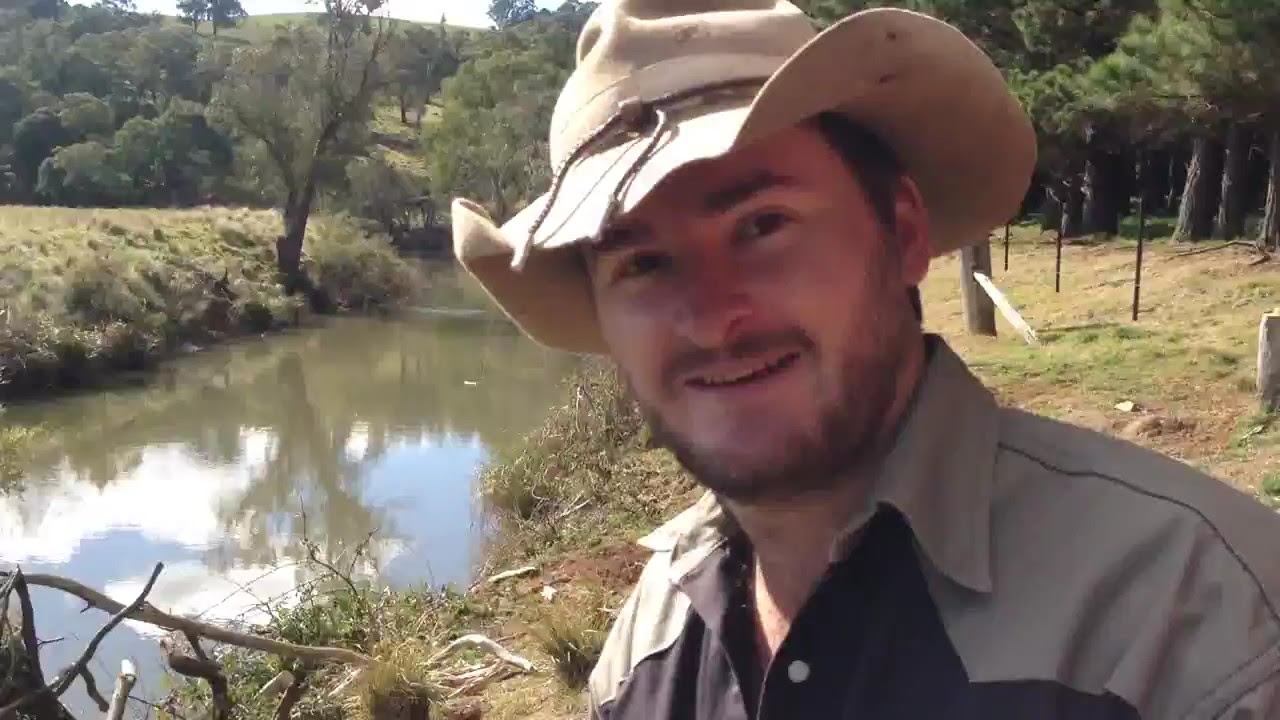A photograph captures a young white man in his 30s, bearded and mustached, looking straight at the camera with a smile. He wears a wide-brimmed khaki hat, reminiscent of Australian bush or cowboy style, and dons a buttoned shirt combining light and dark brown tones. The setting is outdoors in a serene wooded area. Directly behind him lies a still canal or stream, mirroring a blue sky with scattered white clouds. The background features a lush forest filled with green trees, interspersed with some dead branches. Above the man's right shoulder, in the upper-right corner of the image, a few fence posts are visible, enhancing the rustic, natural atmosphere.